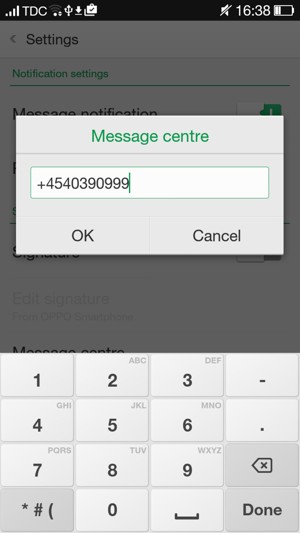The screenshot displays a mobile phone screen with a pop-up notification tab in the center, creating a foggy gray overlay on the top two-thirds of the background. At the very top of the screen, there's a black border featuring several status icons: from left to right, full Wi-Fi signal, a TV icon, and a battery icon which is only a quarter filled in white, indicating partial charge. The time is shown as 16:38, and the sound is muted.

On the left side, partially obscured by the foggy overlay, a "Settings" label is visible, and beneath it in green is "Notification settings". In the background's top half, there's a "Message Notification" label in black, partially visible.

The focal point of the screen is the light blue pop-up tab termed "Message Center" in green text, with a gray horizontal line beneath it. Inside this tab is a white rectangle running almost the full width of the screen, containing a numeric sequence: "+54 454-039-0999." Below this, there are two buttons: "OK" on the left in black and "Cancel" on the right.

In the faded backdrop, "Edit signature" can be slightly discerned. Below this, there's an on-screen keypad with light gray buttons for the numbers one, two, three, and a dash in the first row. The second row has the numbers four, five, six, and a period. The third row contains the numbers seven, eight, nine, and a delete button. The bottom row displays an asterisk, a pound sign, and a partially-visible curved button in light gray, then a zero, and a long space bar with edges pointing upwards. Finally, the word "Done" is written in black on a dark gray button.